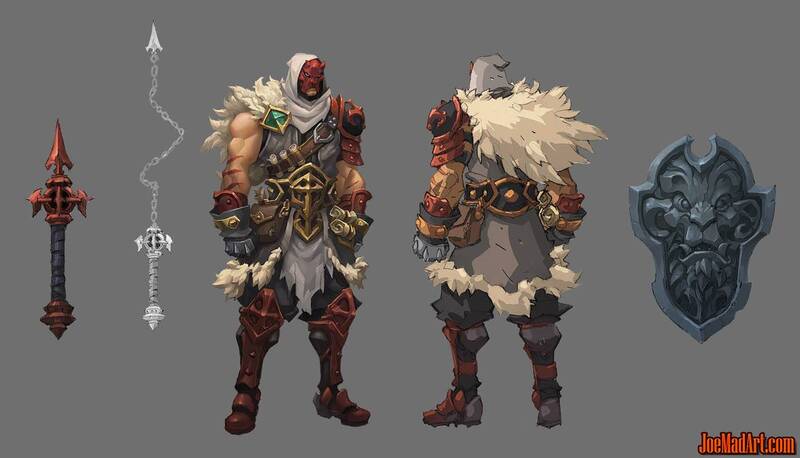This character design concept art, likely created digitally, features a formidable, muscular warrior clad in intricate armor, positioned centrally against a gray backdrop. The character appears twice - a front and back view - showcasing various aspects of his detailed attire and gear. He stands over six feet tall with a brooding presence.

The warrior wears elaborate armor, leaving his right arm fully exposed but protected by a glove and gauntlet, while his left shoulder is shielded with red and black protective gear. His striking facial features are obscured by a devil-like mask with prominent horns, revealing only the lower part of his face. Over the mask, he dons a gray hood adorned with white feathers at the tail. His central armor includes a gun belt across the chest, an armored belt at the waist, and massive red boots.

To the left of the character, the weapons are prominently displayed. One weapon is a red-tipped spear or javelin with a black pole. The other is a complex chain weapon featuring a spiked end, a bludgeoning item, and a clutching device along the chain. On the far right side of the image is the shield concept, designed as a lion's face crafted from a marble-like blue material. The entire artwork is set against a rectangular gray background, with "joemadart.com" visible in orange lettering in the lower right corner.